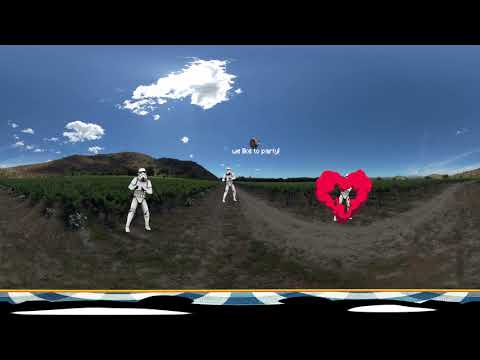This augmented reality scene captured outdoors against a bright blue sky with two large cumulus clouds and the sun partially hidden behind the larger cloud depicts a dynamic setting featuring elements from a video game. At the heart of the image are two stormtroopers—one positioned in the center and the other to the left of the frame. On the right side of the center stormtrooper, there is a conspicuously floating red heart shape, suggesting a possible in-game effect.

The bottom edge of the image presents a distinct border comprised of black bars forming a 16:9 letterbox effect. Within this frame, there is a yellow line and alternating blue and white shapes, giving the impression of a vehicle's dashboard or an interface element. Below this, a dirt path lined with patches of green grass winds through the scene, curving to the left before sharply bending at the right edge of the image. Despite the dynamic composition, the overall setting maintains a serene rural backdrop with a green field and a hill on the horizon. The layered colors in the scene include black, white, gray, blue, green, pink, and yellow, all contributing to the vibrant yet cohesive visual experience.